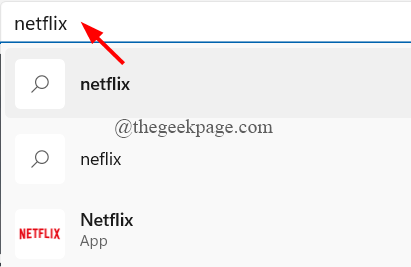The image is a small screenshot displaying a search interface, likely from a website or a mobile application. At the top of the screenshot, there is a search bar where the term "Netflix" has been entered. To the right of the search bar, a red arrow has been manually added to the screenshot, pointing diagonally up and to the left towards the search bar, with a label indicating "Netflix."

Below the search bar, the first search result is highlighted in a darker gray shade and includes an hourglass and magnifying glass icon followed by the word "Netflix." The second search result is similar but is not highlighted, featuring the same icon and the word "Netflix."

Further down, there is a third result showing a small square icon with the red Netflix logo (the word "Netflix" in red), followed by the text "Netflix" and "app" underneath it.

The overall background of the screenshot is predominantly white, with a blue line at the top separating the search bar from the search results. Additionally, there is a watermark in the center of the screenshot reading "thegeekpage.com," suggesting that the screenshot is part of an article or tutorial from the GeekPage website on how to search for Netflix.

This comprehensive description offers a clear visual and contextual understanding of the screenshot, detailing every element present in the image.